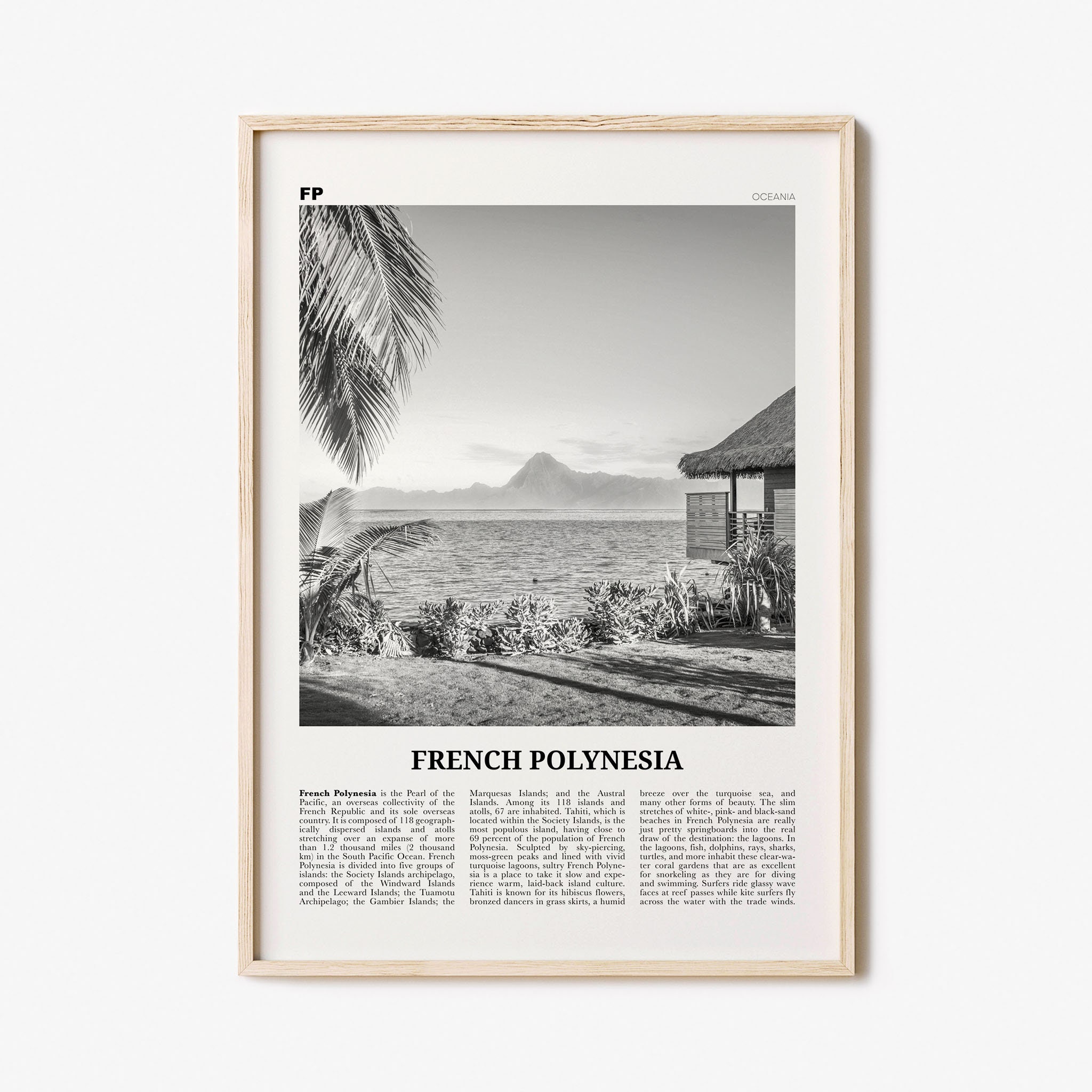A framed magazine page is displayed on a white wall, housed in a light beech wood frame with a raw, unstained finish. At the top left corner of the article, "FP" is printed in bold black letters, while "Oceana" appears in light gray on the top right. Below these headings is a large black-and-white photograph depicting a serene beach scene. This image includes a sandy shore in the top right corner, a hut or shack with palm fronds hanging down on the right, and a picturesque view of an ocean leading toward distant mountains or volcanoes. The photograph is bordered in white. Below it, the title "French Polynesia" is prominently displayed in bold letters, followed by three short columns of text that comprise the main article. The entire setup, from the framing to the content, exudes a sense of nostalgic elegance.